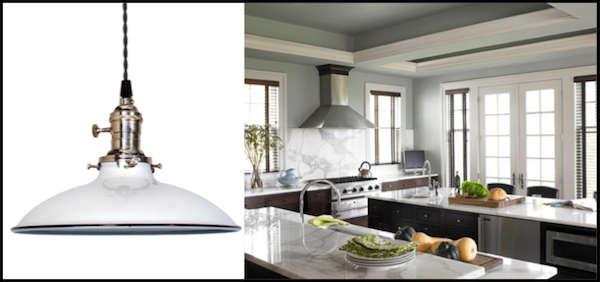The image consists of two sections: the left side features a sleek, modern hanging ceiling light with a white main body and a golden metallic upper part, set against a white background. This pendant light has a stylish design with an upward-extending wire. On the right side, the image showcases an elegant, pristine, and spacious kitchen. The kitchen boasts gray walls and ceiling, a cooktop, a chimney, a washbasin, and an island with a built-in faucet, which doubles as a breakfast counter. The countertops are adorned with a variety of fruits and vegetables, contributing to the kitchen's clean and welcoming atmosphere. The windows offer additional light, enhancing the kitchen's modern and inviting aesthetic.